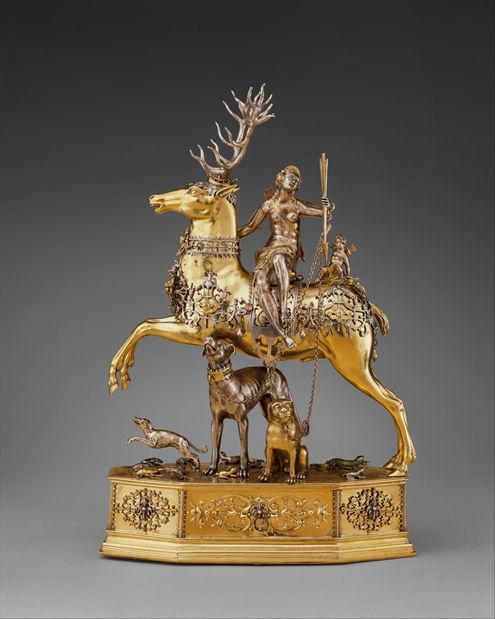A portrait-oriented image captures a gold-finished decorative statue set against a gray gradient background. The ornate base of the statue is an octagonal shape, intricately designed, adding to its grandeur. At the base, a few dogs are depicted in dynamic poses, with chains that connect them and a grand reindeer that dominates the scene above. The reindeer, adorned with decorative elements and impressive antlers, is in mid-prance, with its front legs raised and back legs grounded. Seated sideways atop the reindeer is a topless figure, possibly a woman, gazing upward while holding a stick linked with chains. The attention to detail in the statue emphasizes the elegance and craftsmanship of the piece.